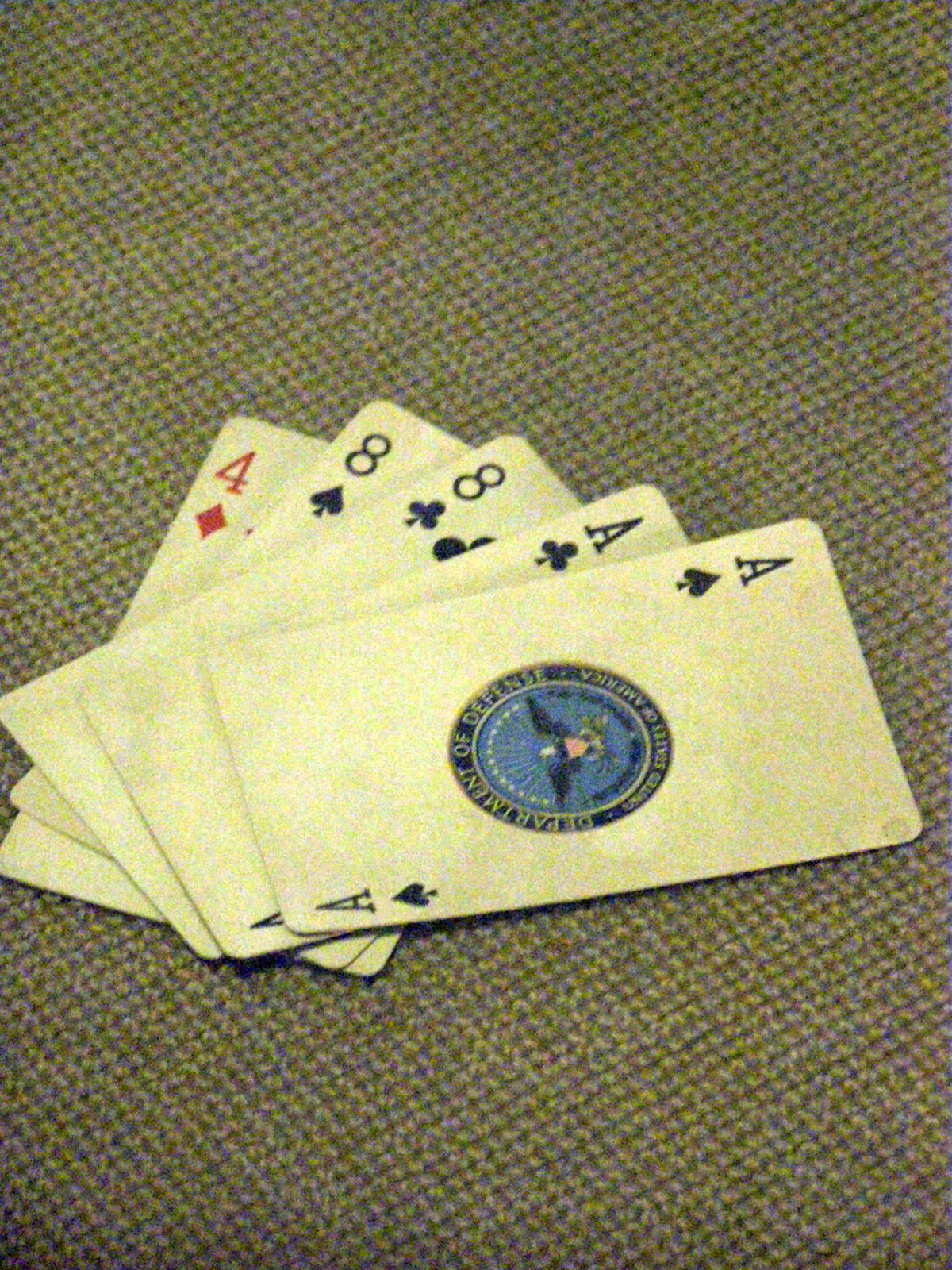The image depicts a set of five standard-sized playing cards elegantly arranged on a textured brown fabric, which could be a tablecloth or a throw. The cards, placed from right to left, include the Ace of Spades, Ace of Clubs, Eight of Clubs, Eight of Spades, and the Four of Diamonds. Together, these cards form the notorious "dead man's hand," a legendary poker hand associated with the death of Wild Bill Hickok, rather than Jesse James.

In the center of these cards lies an insignia featuring the Department of Defense emblem, highlighted by a detailed Bald Eagle at its core. This emblem is prominently placed and serves as a focal point within the arrangement of the cards. The juxtaposition of the historical dead man's hand with the modern insignia of the Department of Defense lends a unique and thought-provoking juxtaposition to an otherwise classic poker hand.